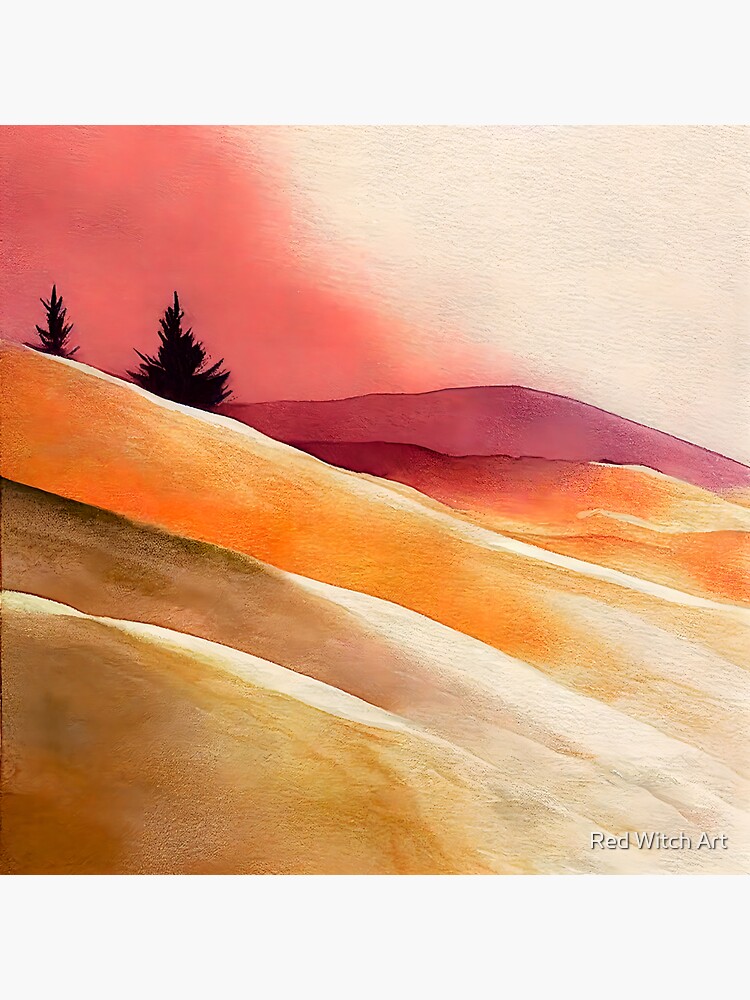This is a square-format watercolor painting depicting a vibrant hillscape, mounted on an off-white wall. The painting features a series of rolling hills and mountains with a striking variety of colors and an abstract style. In the foreground at the bottom left, there are golden-yellow hills with curved ridges highlighted in cream, transitioning into a dark brown section and a lighter orange area above it. Moving towards the middle, there's a dark-purple mountainous terrain on the horizon, accompanied by lower, dark-orange hills in front of it. 

To the left, the tops of two pine trees, rendered in black ink, rise in silhouette. The leftmost tree is only partially visible, while the other is more prominent, situating itself next to a colorful background. The sky to the left is an orange-red hue, blending into pink behind the trees and gradually fading to a cream color on the right side. This seamless gradient enhances the landscape's ethereal quality.

In the bottom right corner, the painting is signed with the text 'Red Witch Art' in a white font with black shadowing, adding a final touch to this captivating piece.